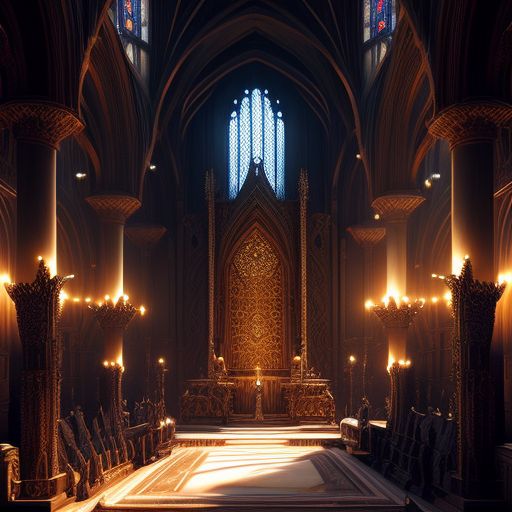The stylized image depicts the interior of a dimly lit, elaborate church-like structure with a tall vaulted ceiling. Dominating the scene are prominent columns and arches that frame the space symmetrically on each side, with smooth, marble-like pillars accented by spiny, cactus-shaped bases. Rising halfway up, these pillars support inverted trapezoid structures that hold up delicate, pointy arches. Stained glass windows with blue and red designs flank both sides of the image, while a brighter, non-colored rectangular window, featuring a curved shape reminiscent of five outstretched fingers, casts a daylight hue at the center top third of the frame.

Central to the composition is an ornate, door-like structure that appears to function as an altar or throne. It features intricate, vine-like designs with what looks like an eye at its center. Flanked by unadorned, pointed pillars, the altar stands atop a richly striped gold and red base. Directly below, a brightly lit walkway extends towards this central focal point, guiding the viewer's eye. Despite the dark ambience of the image—accentuated by brown and orange tones—the interplay of stained glass and subtle lighting from candles enhances the mystical, almost otherworldly atmosphere of this unique, possibly AI-generated interior.